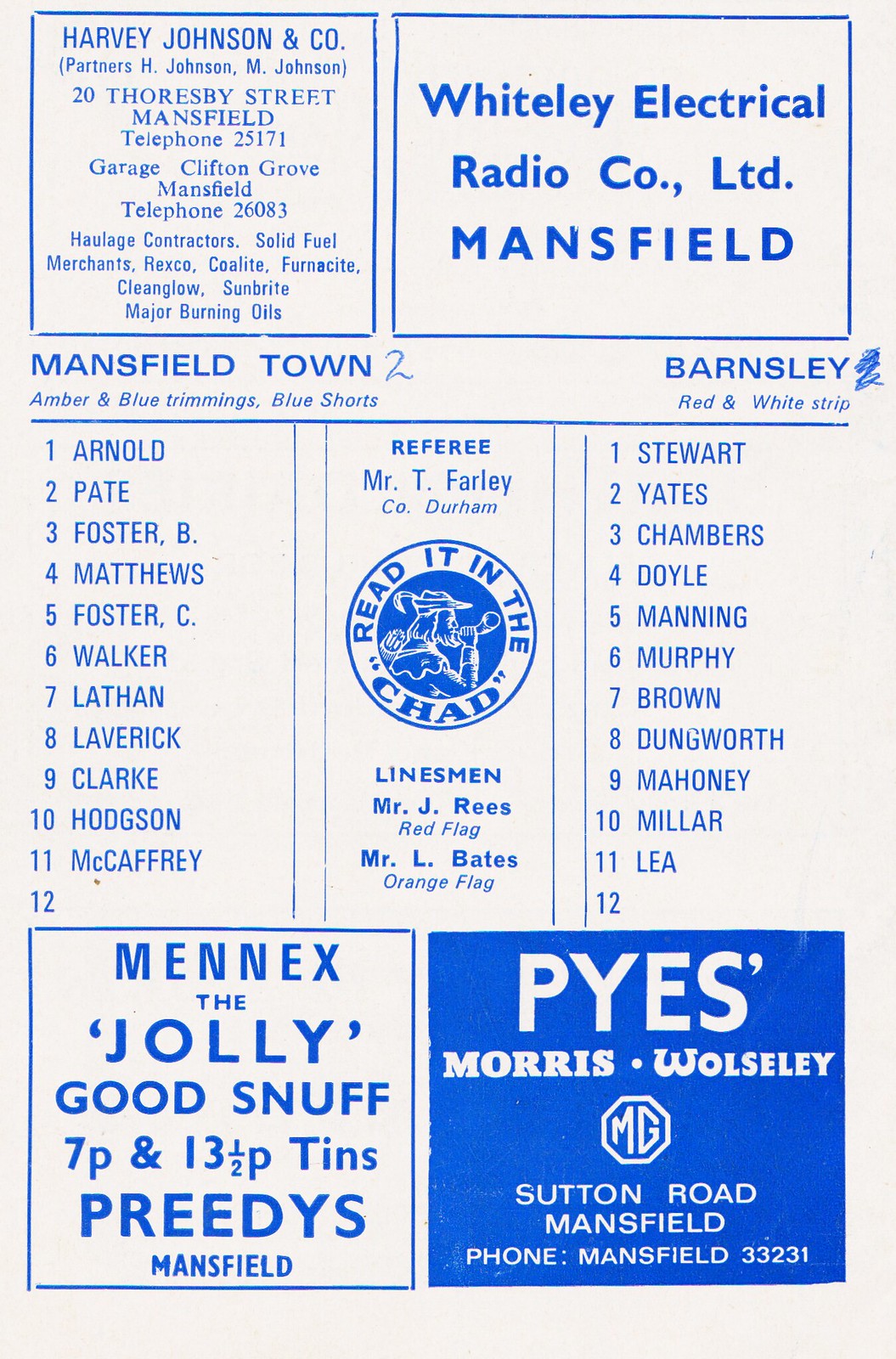The image depicts a page from a sports program, primarily white with blue text. Central to the page is information about a match, detailing "Mansfield Town 2" versus "Barnsley." Mansfield Town's colors are mentioned as having amber and blue trimmings with blue shorts, while Barnsley's colors feature red and white stripes. Both teams' player lists are numbered from one through eleven. 

In the upper left corner, there are advertisements including Harvey Johnson & Company, which is a garage and solid fuel merchant located at Clifton Grove, Mansfield, with a contact number of 26083. Other ads in the left margin feature Whiteley Electrical Radio Company Limited from Mansfield and Menex, advertising "The Jolly Good Snuff" in 7p and 13.5p tins.

The bottom portion has more advertisements, including one for Pies Morris and Wolsley MG, located on Sutton Road, Mansfield with a phone number of 33231. Centrally, it lists match officials: Referee Mr. T. Farley, and linesmen Mr. J. Reese holding the red flag and Mr. L. Bates the orange flag.

Overall, the image combines detailed information about the ongoing sports event and various local advertisements, all framed with blue text on a white background.